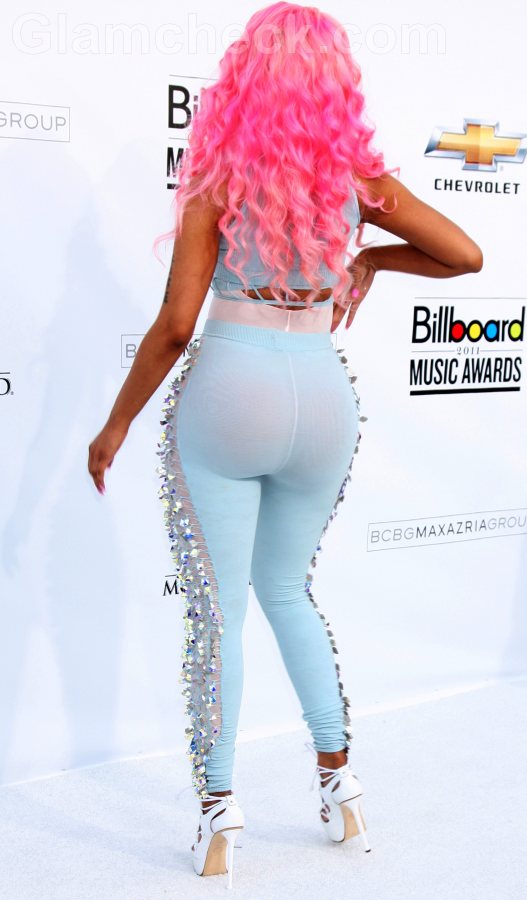In this vibrant color photograph, a woman with a darker skin complexion is captured from behind as she faces a backdrop of a white wall adorned with logos and text. She sports bright, voluminous pink curly hair, which cascades down her back. She is dressed in a light blue tank top layered over a white one, paired with matching light blue leggings embellished with sequins running along the sides. Her ensemble is completed with white high-heeled shoes and bright pink nails that stand out. Her right arm is raised slightly, while her left arm hangs straight down. The backdrop prominently features the text "Billboard Music Awards," the Chevrolet logo in gold, silver, and black, and partially visible text "BCBGMAXAZRIAGROU." The setting appears to be a red carpet event, suggested by the mentions of a red carpet and the award show backdrop. Overall, the image is bright, likely due to natural light, and places the woman as the focal point without any other individuals in sight.